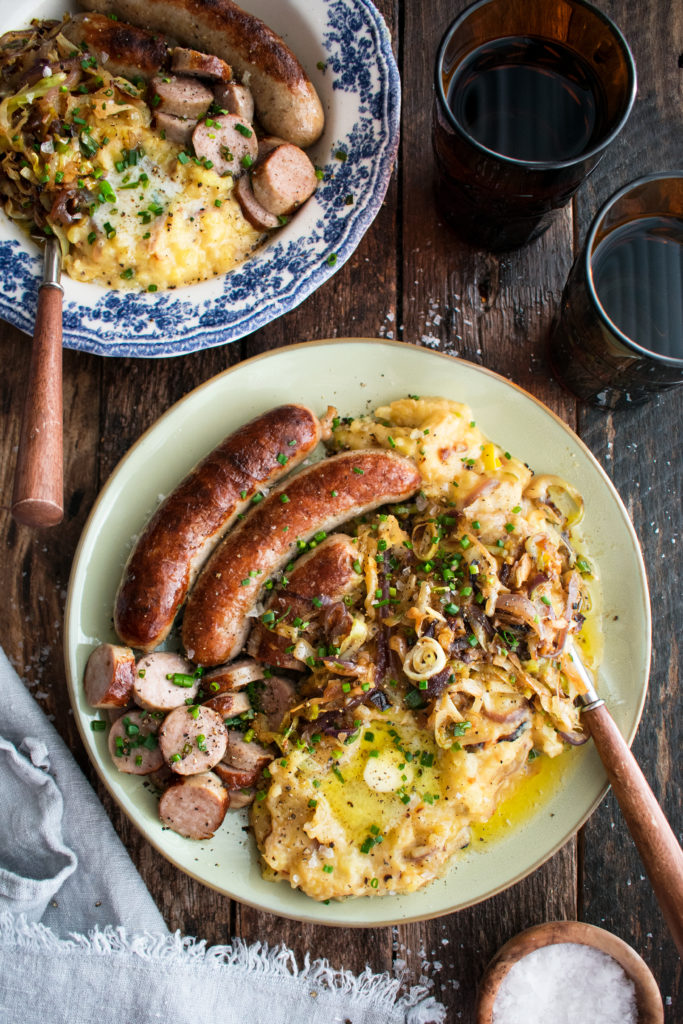The image depicts a top-down view of a rustic, weathered wooden table with a dark brown finish. In the upper right corner, there are two amber glasses filled with a dark liquid. On the table, there are two plates: one is a white porcelain plate adorned with a blue floral pattern around the rim, while the other plate has a combination of colors, appearing mostly white with gold detailing. Both plates contain a mix of food, including two whole sausages, sliced sausages, and a starchy, buttery dish that looks like mashed potatoes mixed with onions and possibly some chicken stew. Both dishes have wooden utensils submerged in the food, making it difficult to identify whether they are spoons or forks. Additionally, there's a small wooden bowl containing a white, powdery substance, likely salt, placed at the bottom right of the image. In the bottom left, there is a neatly folded white towel. This detailed setting suggests a hearty, rustic meal ready for enjoyment.